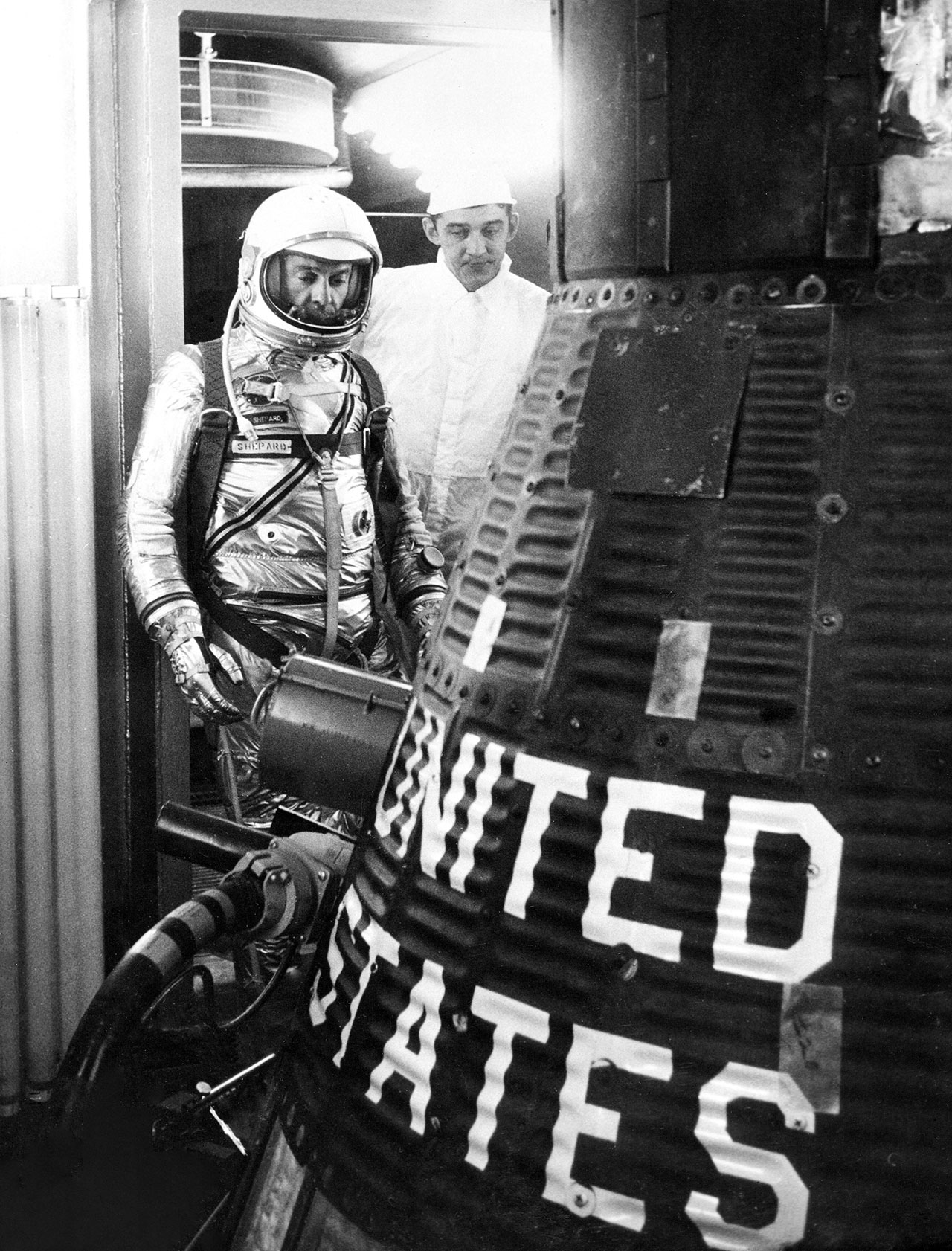The photograph is a detailed black-and-white image from the 1960s, capturing a NASA space command module prominently labeled with "United States" in large white letters near its base. The module itself is a solid black, conically shaped structure with enriched, ribbed paneling that gives it a corrugated appearance. An astronaut, identified by the name tag "Shepard," stands in front of the space capsule. Shepard is clad in a silver, reflective spacesuit with a white helmet and visor, and a backpack on his back. Beside him, to his left, stands another person in clean white attire, resembling a clean room suit, observing the space module with him.